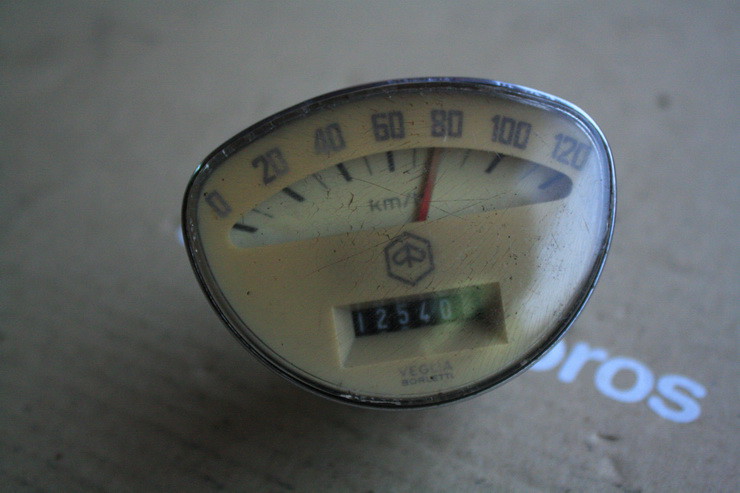This photograph showcases an oval-shaped speedometer and mileage counter, typically extracted from an automobile. The speed readings are calibrated in kilometers per hour, ranging from 0 to 120 km/h. Black numbers mark the speed increments, set against an off-white background. The needle, which moves to indicate speed, is red. The entire instrument is encased in a silver surround, enhancing its polished look. The device rests on a cardboard surface, which features partially visible white lettering, including "R-O-S." Additionally, there is a visible mileage reading of 12540, although the last digit is obscured. The manufacturer's branding, partially visible, reads "VEGIA" followed by something resembling "Boroleti." This speedometer and mileage counter unit appears to be an authentic automobile part, likely removed for either display or repair.